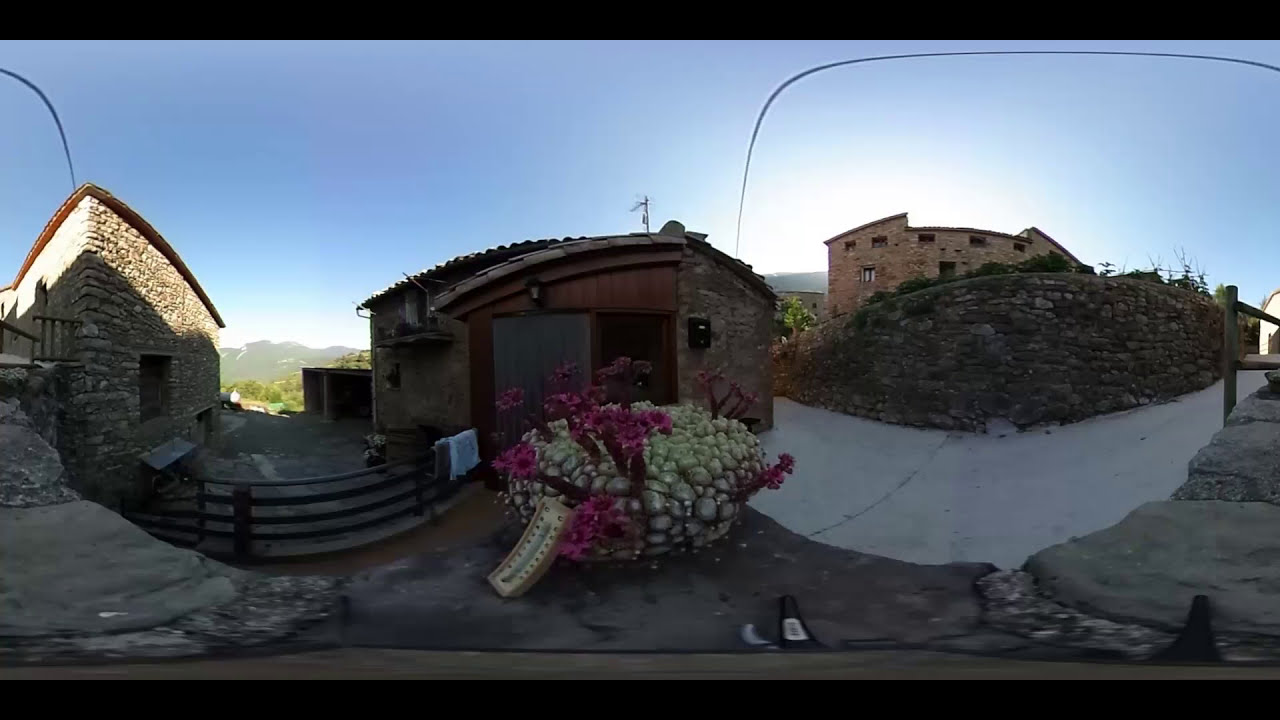The photograph is a horizontally oriented, panoramic outdoor image taken with an unusually distorted lens, resulting in a curvature effect throughout the scene. Dominated by a bright blue sky above, the image below reveals a dark, shaded area. There are three small buildings made of stone, with curved and slightly lopsided roofs, that contribute to a quaint, rustic atmosphere. In the foreground, a large planter or a bundle of flowers with pink blooms is prominently featured, with an outdoor thermometer leaning against it. A stone wall runs alongside a paved path or concrete driveway leading towards these buildings. A low wooden fence separates the buildings from a section of bare ground. On the right side, another house appears in the background, with a curved fence adding to the lens-induced distortion. Additionally, a large gray boulder is situated in the lower right quadrant of the image. The entire scene is bathed in the bright sunlight of a clear day, highlighting the contrasting textures and curvature of the distorted landscape.